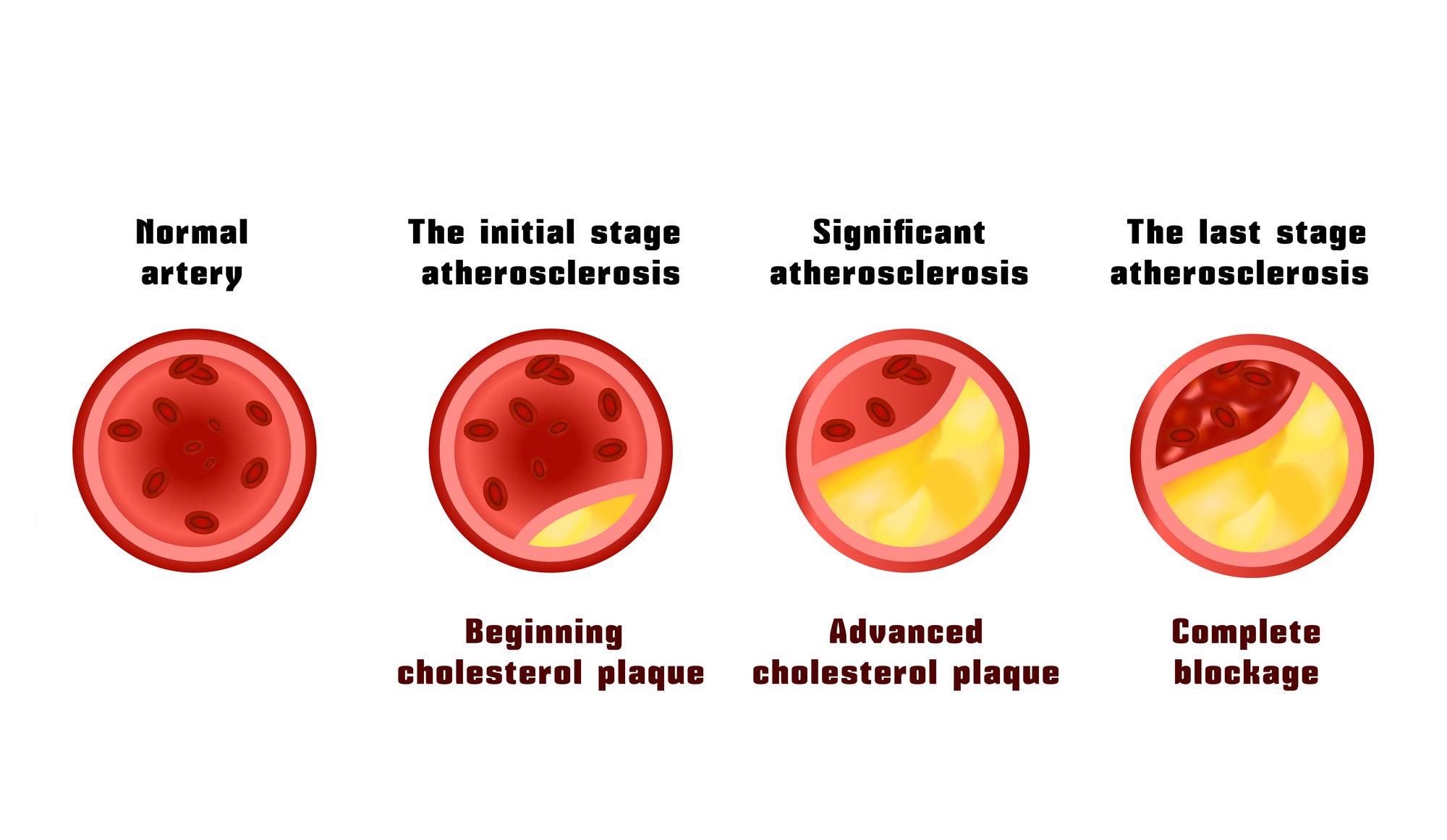The image is a medical chart consisting of a series of animated circles, representing the progressive stages of artery blockage due to arteriosclerosis and cholesterol plaque buildup. The background is white, enhancing the focus on the horizontal row of circles. Each circle shows a cross-section of an artery with varying levels of cholesterol deposits:

1. The first circle, labeled "Normal artery," illustrates a healthy artery with a red outer lining and a pink inner lining, filled with red blood cells.
2. The second circle, "Initial stage: Beginning cholesterol plaque," shows the artery starting to fill with a yellow substance in the lower right corner, signifying the early accumulation of cholesterol.
3. The third circle, "Significant arteriosclerosis: Advanced cholesterol plaque," depicts the artery more than half-filled with yellow cholesterol deposits, reducing the flow of red blood cells.
4. The final circle, "Arteriosclerosis: Complete blockage," demonstrates an almost completely obstructed artery. Only a small portion remains visible in dark red, heavily packed with smaller red dots, indicating severe blockage.

Each stage visually contrasts with the previous one by the increasing presence of yellow cholesterol and diminishing space for red blood cells, depicting the artery's progression towards complete occlusion.